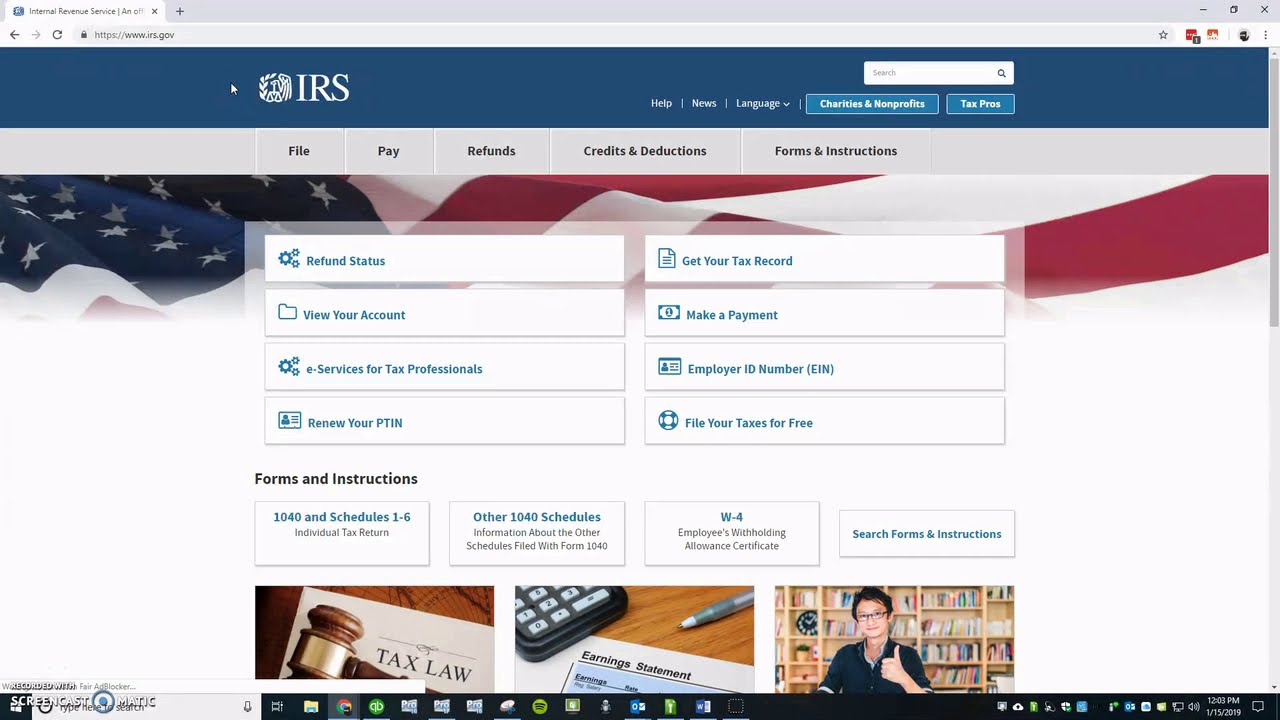This image shows the detailed layout of the IRS Internal Revenue Service website's landing page. At the very top, a navy blue ribbon prominently features the white IRS logo on the left. To the right, there are accessible options for "Help," "News," and "Language." Below this, a light blue box labeled "Charities and Non-Profits" is positioned next to another box for "Tax Pros," above which lies a white search bar for quick navigation.

Directly beneath these elements, a light gray ribbon offers crucial links including "File," "Pay," "Refunds," "Credits and Deductions," and "Forms and Instructions." The main content is divided into two vertical columns of options starting from the top left: "Refund Status," "View Your Account," "E-Services for Tax Professionals," and "Renew Your PTIN." In the adjacent column, the options include "Get Your Tax Record," "Make a Payment," "Employer ID Number (EIN)," and "File Your Taxes for Free."

Further down the page, additional links are organized into categories such as "Forms and Instructions," including "1040 and Schedules 1 to 6," "Individual Tax Returns," "Other 1040 Schedules," and "W-4," along with a search function for more forms. Towards the bottom, the page features several images that are unfortunately cut off midway, hinting at more visual content or links that extend beyond the visible area.